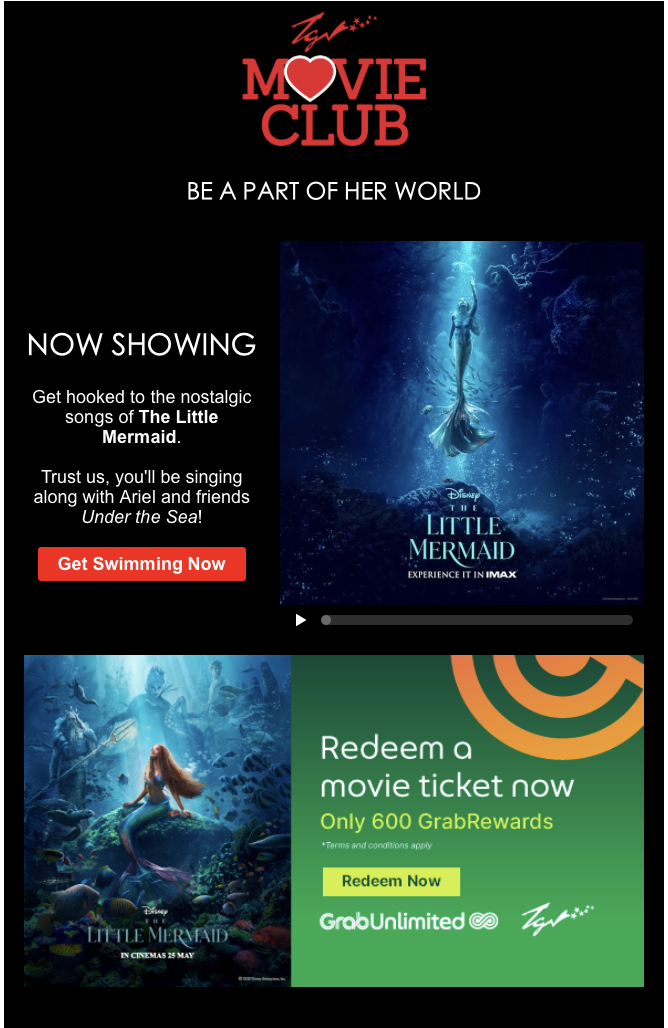The image appears to be a promotional advertisement for a Disney movie club featuring "The Little Mermaid." At the top, an illegible signature, possibly "Taylor," is scribbled in red. Beneath it, the text "Movie Club" is prominently displayed in red font, with a heart symbol replacing the 'O' in "Movie." Accompanying this, the slogan "Be a part of her world" is written in smaller white letters. Below this, further text in white reads: "Now showing, get hooked to the nostalgic songs of The Little Mermaid. Trust us, you'll be singing along with Ariel and friends under the sea."

To the right of this text, there is a promotional image from the movie featuring Ariel, the Little Mermaid, swimming towards the surface in a beam of light. Below, another poster depicts Ariel sitting on a rock with her red hair flowing behind her, along with her father and friends like Sebastian in the background.

Adjacent to this lower poster, in a green box, the advertisement encourages viewers to redeem a movie ticket: "Redeem a movie ticket now, only 600 grab rewards," with a yellow button labeled "Redeem Now, Grab Unlimited." The same scribbled signature appears again in white in this section.